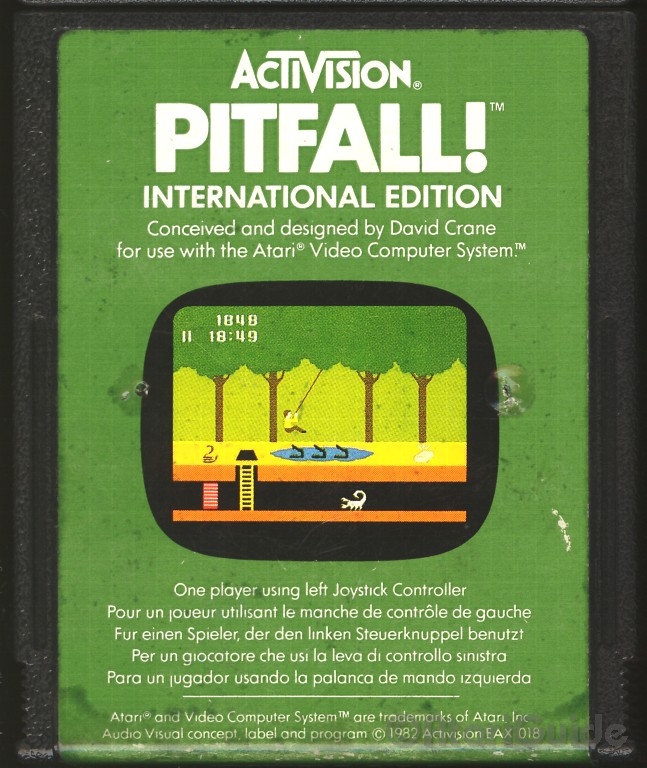This image features the cover of a vintage video game, prominently displaying a green background with a black border. The cover's rectangular shape, taller than it is wide, is closely cropped and contains a centered text and image layout. The title "Pitfall!" in bold white text stands out, followed by "International Edition" underneath. Beneath this, it declares that the game was conceived and designed by David Crane specifically for use with the Atari video computer system, a reminder further emphasized by noting that Atari and the video computer system are trademarks of Atari Inc. Additional text indicates details such as "One player using left joystick controller" and lists the audio-visual concept label and program from 1982 by Activision, labeled as EAX018.

In the middle of the cover, a vintage television-shaped graphic showcases a screenshot from the game depicting a classic woodland scene. The scene includes green trees, a person swinging on a rope over a pool, a nearby ladder, and a scorpion, all within a vivid rectangular frame. The presentation and multilingual details underscore the "International Edition" aspect of this iconic game.